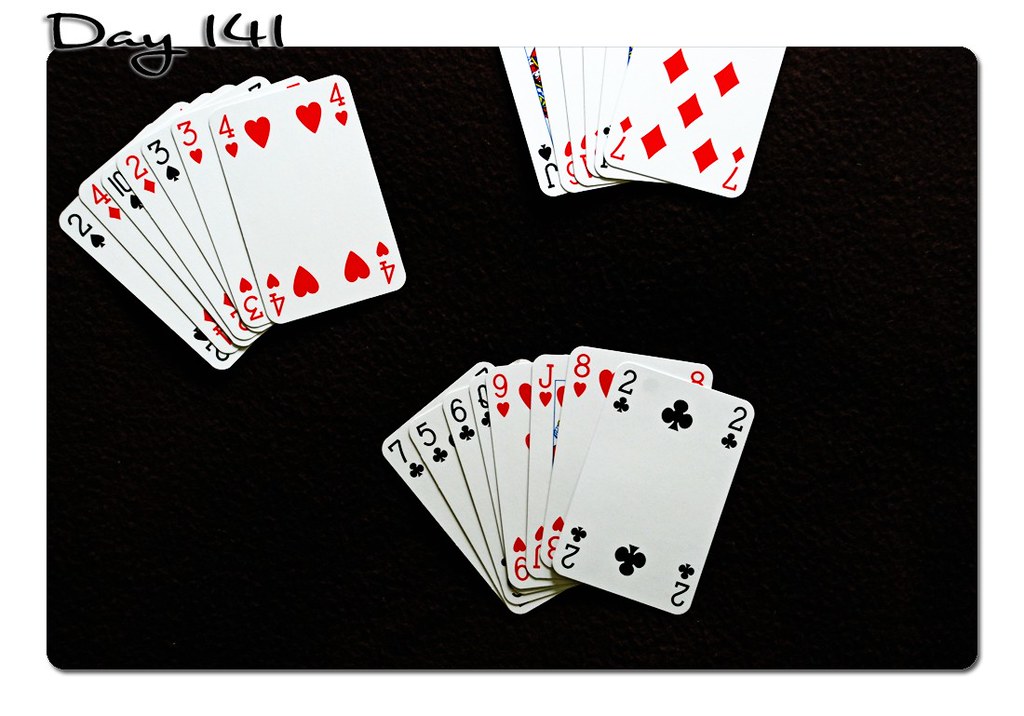The image features a complex card layout set against a solid black background, creating a dramatic and focused display. At the bottom of the screen, seven visible playing cards are neatly arranged in the following order: 7 of clubs, 5 of diamonds, 6 of spades, Queen of clubs, 9 of diamonds, Jack of hearts, 8 of hearts, and 2 of clubs. In the top left quadrant, a cluster of seven more cards is discernible: 2 of spades, 4 of diamonds, 10 of spades, 2 of diamonds, 3 of spades, 3 of hearts, and 4 of hearts. At the top center, a smaller hand features cards placed face down with only a few visible: the 7 of diamonds is prominent, followed by hints of cards in a black suit, a red suit, and finally, the Jack of spades. The only text in the image, “Day 141,” suggests this could be part of a long-term playing card game or project. The strategic placement and variety of cards hint at a game more intricate than poker, inviting speculation and interest.